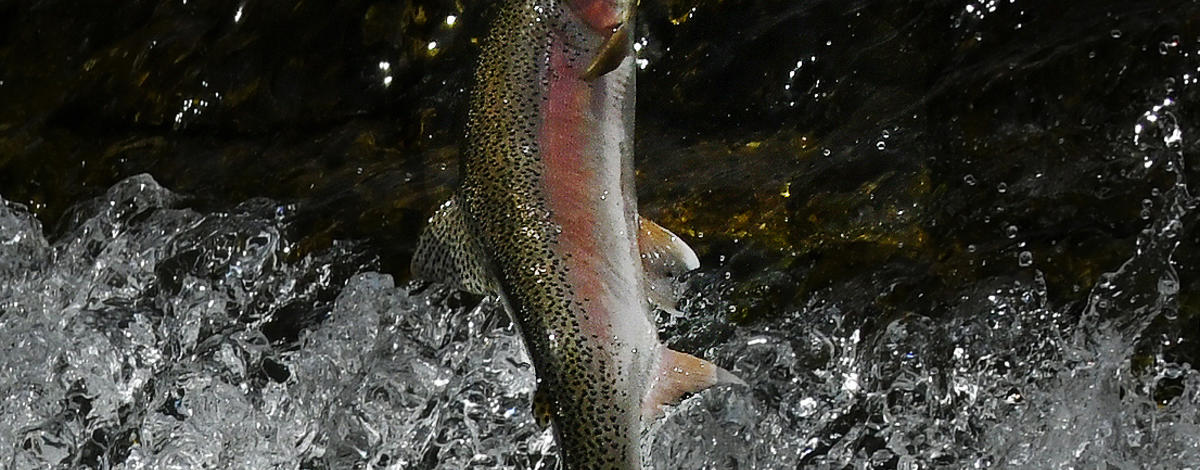This photograph captures a striking image of a salmon leaping out of a choppy stream, throwing up crystalline splashes that shimmer against the dark, likely nighttime, background. The image focuses on about 80% of the salmon's body, omitting its head and tail due to the wide frame of the shot. The salmon itself displays a striking coloration: a pinkish-red center, a greenish top speckled with black spots, and a white underbelly. The fish's midsection is prominent, featuring small fins on the sides and a partially visible dorsal fin. The water below and around the fish appears turbulent, with waves breaking and water droplets suspended mid-air, adding a dynamic, almost painted feel to this vivid capture.